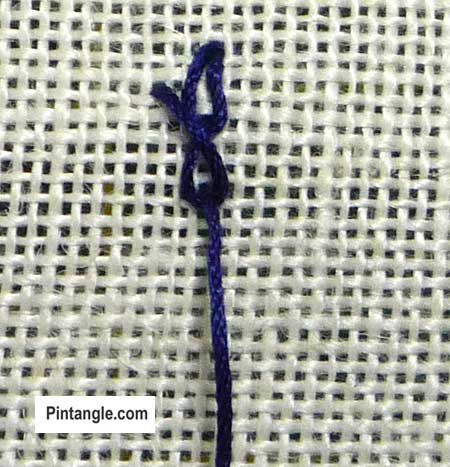The image is a detailed close-up of a loose-weave, white crochet or needlepoint fabric, forming a fuzzy grid with visible square holes. Embedded within this grid is a dark navy blue, almost purple, thread. This thick, yarn-like thread is prominently featured in the center of the image, tied into a knot that forms a figure-eight loop, possibly indicating the starting point of a sewing or stitching project. The backdrop suggests an arts and crafts setting, with a subtle hint of yellow behind the grid. Positioned unobtrusively in the bottom left corner is a small white rectangle displaying the text "pintangle.com" in black font. The thread is slightly off-center to the left, beautifully contrasted against the white fabric grid, which dominates the entire frame.